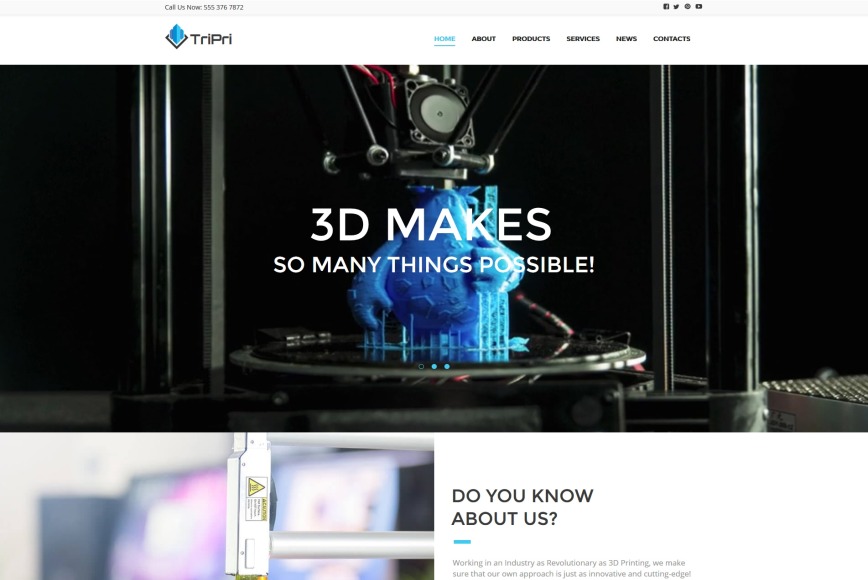This is a screenshot of the TriPri website. At the top of the image, there is a small font text that reads, "Call Us Now, 555-376-7872", accompanied by social media icons for Facebook, Twitter, Instagram, and Snapchat on the right side of the same line. Below this, the TriPri logo is prominently displayed, featuring a blue shape with a black diamond underneath it. The navigation menu is located next to the logo, with options labeled Home (highlighted in light blue), About, Products, Services, News, and Contacts.

The main image spans the width of the website, covering approximately two-thirds of the page. This section features a caption that says, "3D makes so many things possible," and includes a picture of a 3D printer in action, producing a blue-colored object. Below this, a smaller image showcases a detailed, zoomed-in view of the 3D printer, accompanied by the text, "Do You Know About Us? Working in an industry as revolutionary as 3D printing, we make sure that our own approach is just as innovative and cutting-edge."